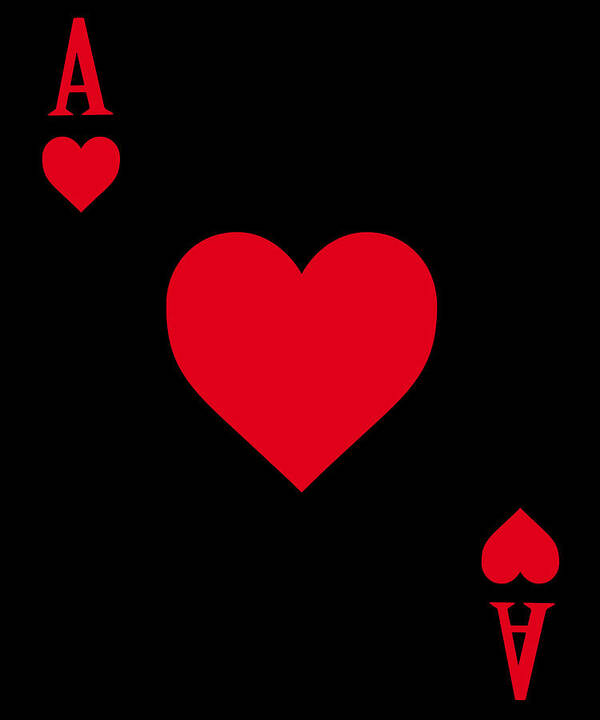The photograph depicts a distinctive ace of hearts playing card set against an all-black background. This card features a traditional yet eye-catching design with red elements. At the top left corner, there's a small upright red heart with a red "A" above it. Meanwhile, the bottom right corner mirrors this arrangement but in an inverted manner, with the heart and "A" both turned upside down. Dominating the center of the card is a large, upright red heart, drawing most of the viewer's attention. The simplified but bold color scheme and the unusual inverted symbols make this ace of hearts stand out against the typical white-background playing cards.